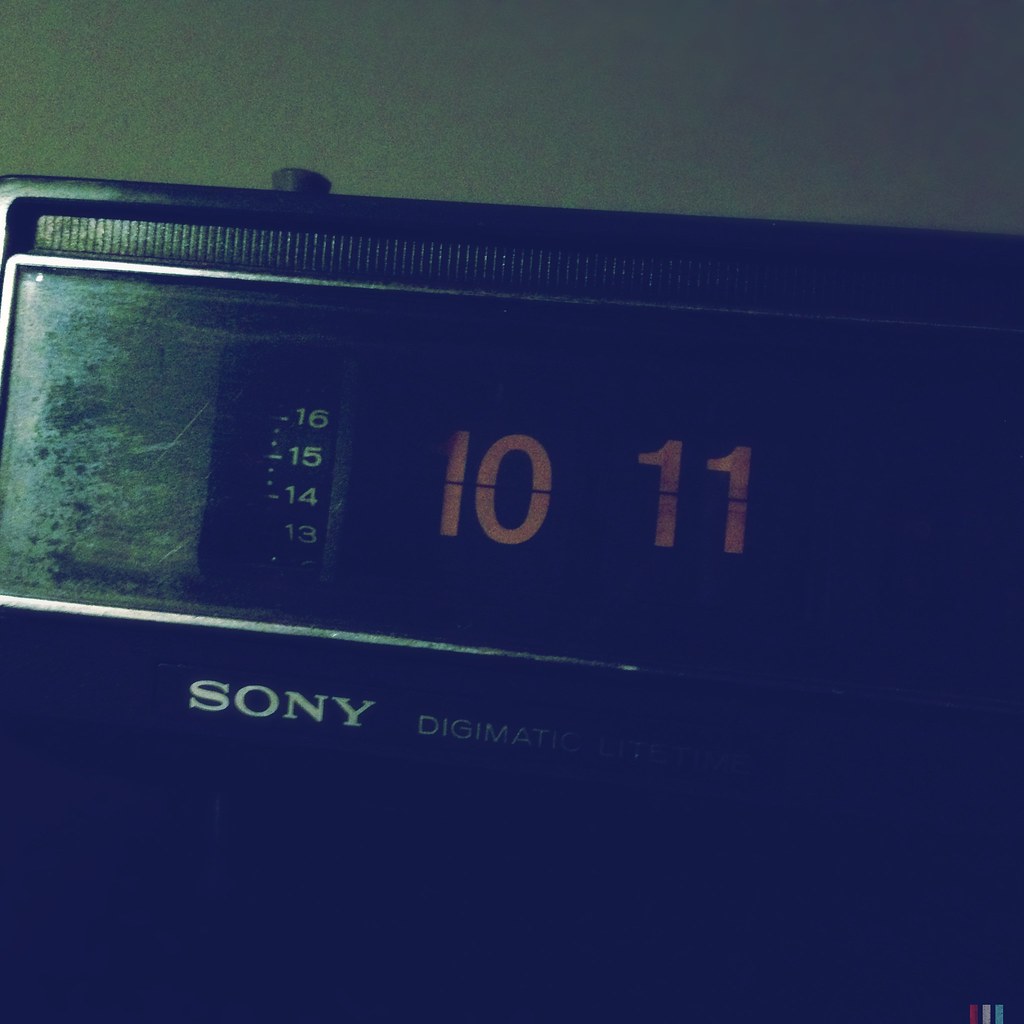This image features a vintage digital clock, presumably from the 1980s, with a classic black plastic exterior. The clock prominently displays the time "10:11" and exhibits signs of wear indicative of its age. Manufactured by Sony, the clock is labeled with the brand name and the model name "Digimatic." Despite some surface scratches on the clear plastic cover and minor paint loss on the digital numbers, the clock retains a nostalgic charm. Adjacent to the digital time display are additional numbers, 16, 15, 14, etc., which could serve either as a radio dial or time adjustment controls. The backdrop of the image includes a gray-toned wall, further highlighting the retro aesthetic of this well-used timepiece.